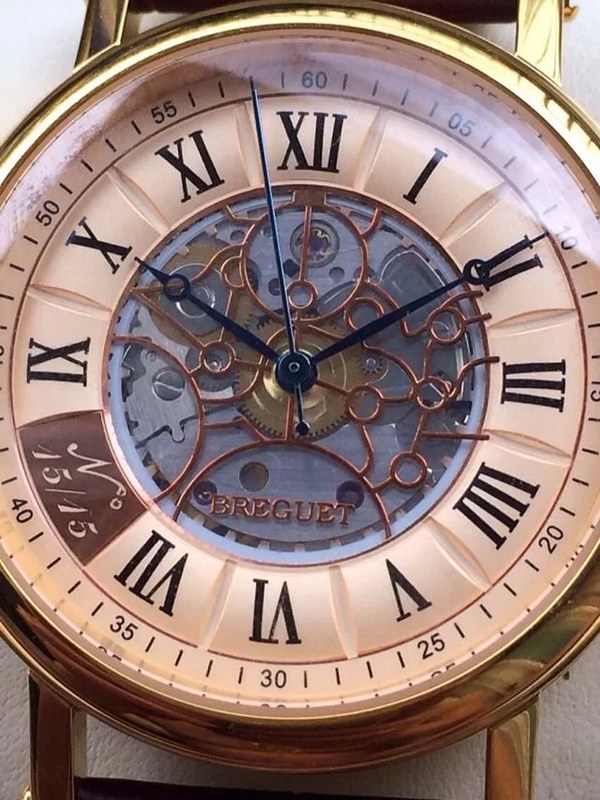In this detailed close-up photograph of a Breguet watch face, the intricate design and craftsmanship are vividly captured. The hands and dials are prominently displayed, showcasing the hour hand positioned at 10 and the minute hand at 2. The watch face features Roman numerals for the hours and additional minute markers encircling the edge. Notably, a small, elegant inscription "N 15/15" is visible on the bottom left side of the face, adding a unique touch to the timepiece. The combination of precision and artistry is evident in every detail of this Breguet watch.